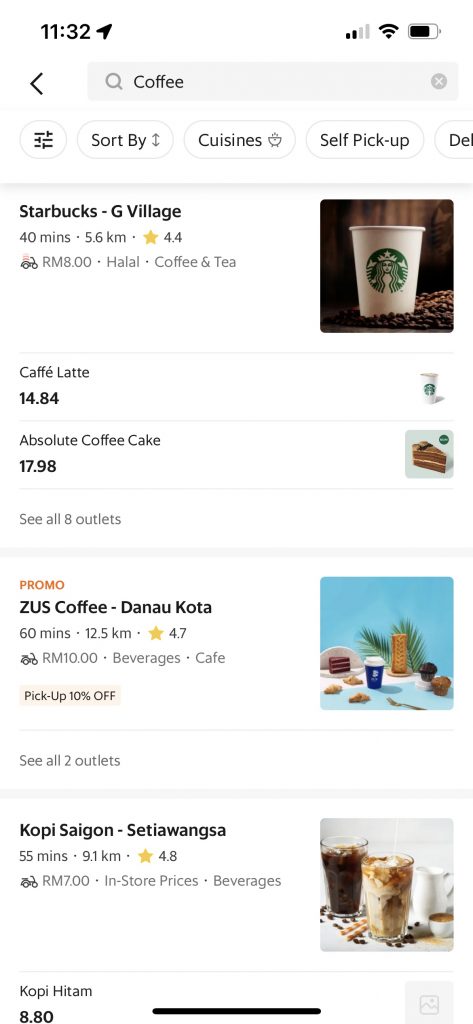In the screenshot of the cell phone display, the time is shown as 11:32, with a location icon nearby. To the right, there are icons indicating cellular signal strength, Wi-Fi connection, and battery life. Below these, there's a search bar with the word "coffee." Following this, there are filters labeled "Sort by cuisine," "Self-pickup," and "Delivery."

The first listing is for "Starbucks-G Village," which is 40 minutes away. The restaurant has a 4.4-star rating. There is also a tricycle icon with "RM8.00," indicating the delivery fee. The listing includes HALAL certification and tags for "COFFEE & TEA." A thumbnail image of a strawberry coffee cup is displayed to the right of this information. Below this listing, items such as "Cafe Latte" priced at RM14.84 and "Absolute Coffee Cake" priced at RM17.98 are shown, each accompanied by thumbnail images. At the bottom, there is a link to "See all eight outlets" in gray text followed by a thin, horizontal light gray line.

The next section is labeled "PROMO," featuring "ZUSCOFFEE DENAU COTA," with details indicating a 16-minute distance over 12.5 kilometers and a 4.7-star rating. A picture icon is also included, along with a link to "See all two outlets."

The final listing is for "COFFEE SAIGON at SETI WANGA SA," which is 55 minutes away, covering 9.1 kilometers, and having a 4.8-star rating. This listing includes a thumbnail image of two beverages positioned to the right.